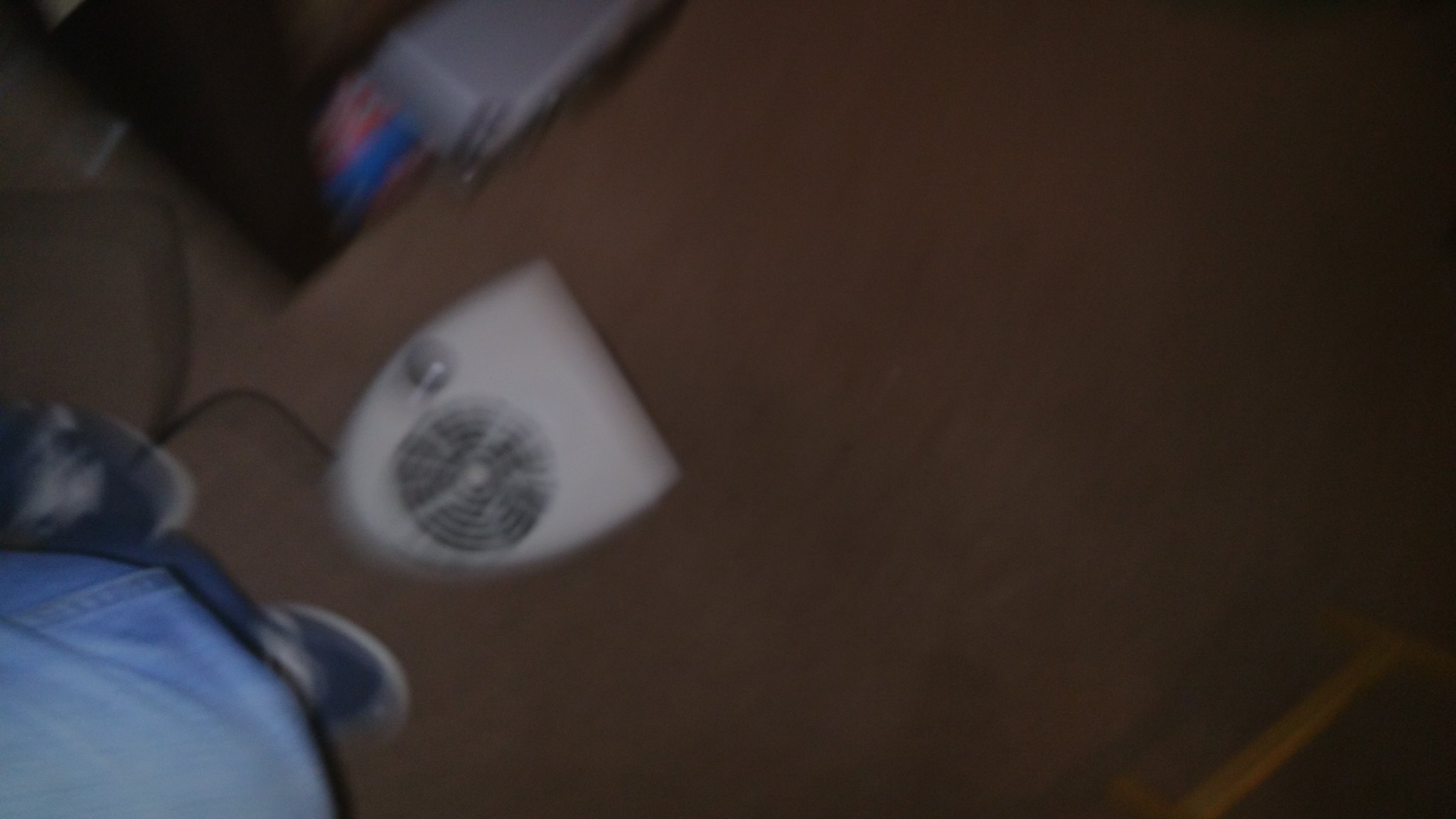In this image, the scene is slightly blurred but predominantly features a brown floor that takes up most of the background. In the top left corner, there's a gray rectangle accompanied by red and blue items, with a dark, almost black, object behind them. In front of these items sits a white device that is flat at the bottom and curves at the top, reminiscent of an oval. This device features two circular vents in the middle, resembling a fan, and also has a silver knob on the left side. Extending from the white object is a black cord. On the left side of the image, there's an object that appears to be made of denim, likely part of a person's blue jeans, and possibly their blue shoe or the pad they are standing on. Near the blurred section, there might also be a brown box underneath the gray one, and silver pads on the floor, suggesting this could be some sort of fan or device operated with foot pedals.